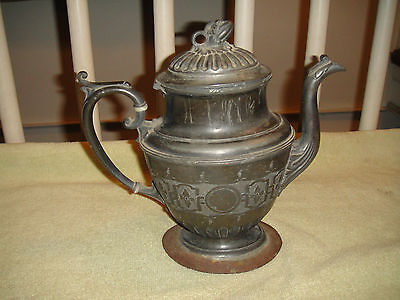The image showcases an antique, possibly silver teapot that appears notably tarnished and in need of polishing. The teapot is adorned with intricate carvings and detailed etchings, particularly prominent on the lid and around the body. The base of the teapot is round, and there is a distinctive band of detailed patterns encircling its middle. The neck of the teapot, designed to resemble a bird's head and body, adds a unique touch to its ornate design. The teapot features several design elements, including circular motifs and shield-like decorations with triangular patterns. It's placed on a pale yellow surface, likely a soft felt blanket or towel. In the background, blurred crib railings fan out and cast shadows on the wall, adding a layered depth to the composition. Light reflects subtly off the teapot, giving it a faint highlight amidst the otherwise muted and flat color palette of bronze, gold, and cream tones.